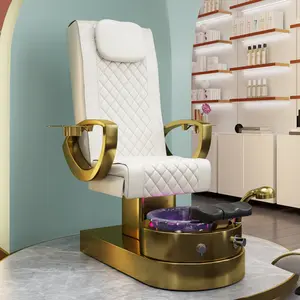The photograph shows an ornate, retro-style salon chair crafted with plush white leather, featuring a high back adorned with a crisscross padded pattern, and a head cushion attached at the top. This chair has sturdy and thick gold (possibly brass) handles and a matching gold base, possibly from the 1950s, that includes footrests and a small black leather platform for soaking feet, indicating it might serve as a pedicure chair. Additional detailing includes a shiny brass ashtray, which enhances its vintage aesthetic. The chair is situated on a gray mat, set against a teal-colored wall. To the right, there is an archway leading to another room and white wooden shelves with red trims lit by fluorescent lights, displaying neatly arranged salon products. The scene is further set within a clean, hip salon environment.